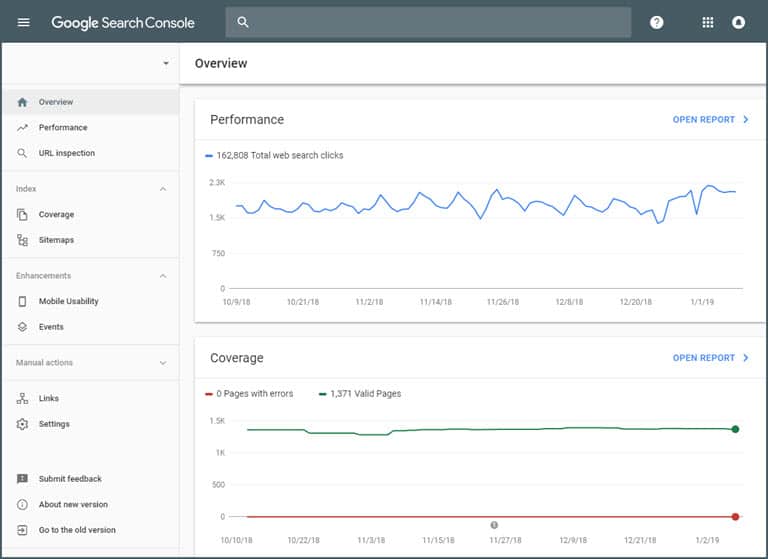This image is a detailed screenshot of the Google Search Console interface. At the top left corner, the title "Google Search Console" is prominently displayed, indicating that this is a tool for managing and analyzing website performance within Google's search engine. The layout, characteristic of Google's design, features a sidebar on the left with various sections including Overview, Performance, URL Inspection, Coverage, Sitemaps, Mobile Usability, Events, Links, Settings, Submit Feedback, About New Version, and Go to Old Version.

In the main section of the interface, two distinct graphs are visible. The first graph, labeled "Performance," is accompanied by a blue-highlighted button at the upper right corner labeled "Open Report." This graph quantifies data with a prominent figure of 162,808 total search clicks.

Beneath the performance graph, there is a "Coverage" graph depicted as a line chart. This section indicates key statistics regarding webpage indexing status, documenting zero pages with errors and 1,371 valid pages.

Overall, this screenshot illustrates comprehensive analytics related to website performance and indexing status on Google's search engine, providing vital tools and insights for webmasters to optimize their sites' search visibility and usability.